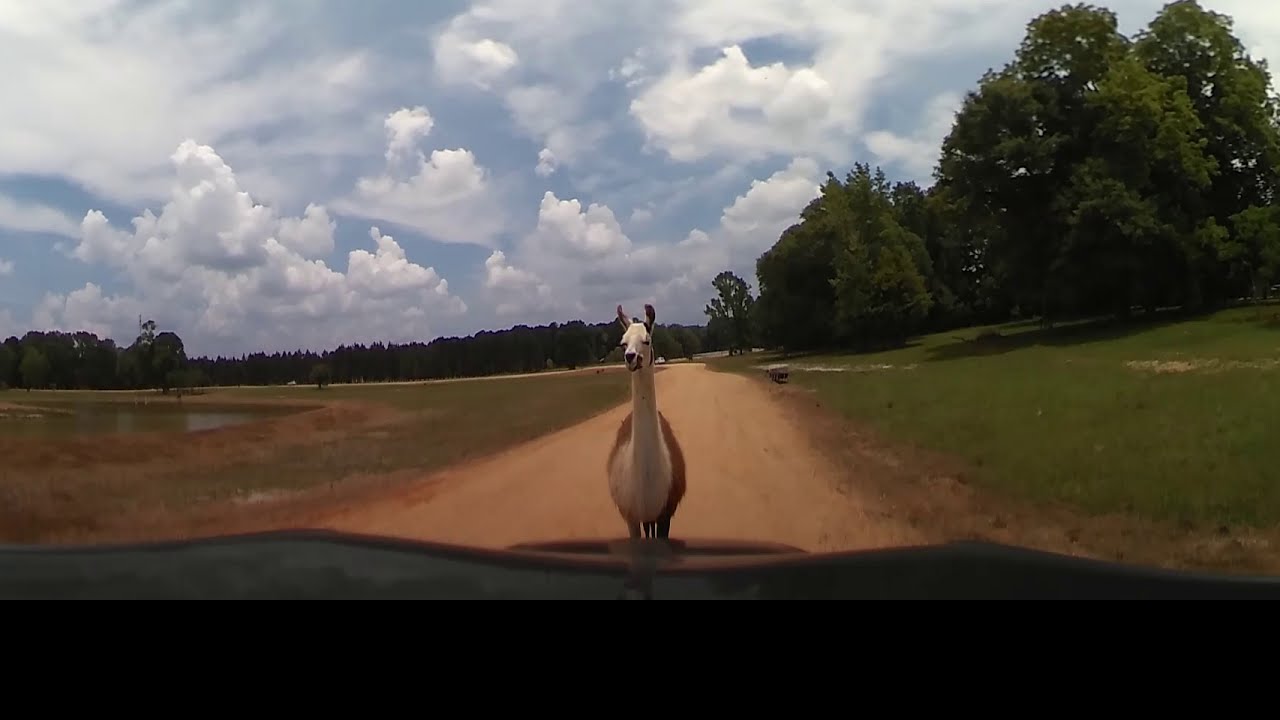The image depicts an outdoor scene taken from a vehicle, possibly a dashboard cam, showing the front of the automobile on a tan, brown dirt road in a park setting. Dominating the foreground is a white llama with a brown body and darker ears, standing directly in the middle of the dirt road and blocking the path. It has a curious expression and distinctive features like a white neck and large, white ears. Surrounding the llama, the landscape includes patches of dry, tan grass along the dirt road, transitioning into greener grass around a small pond on the left. The grassy area around the pond is encircled by trees, which extend into a forested area in the background. The right side of the image features more grassy fields and tall trees. Above, the sky is mostly cloudy with dispersed patches of blue, suggesting daylight conditions. The overall scene captures a tranquil park environment, balanced by the llama's amusing presence and the natural elements of grass, trees, and water.